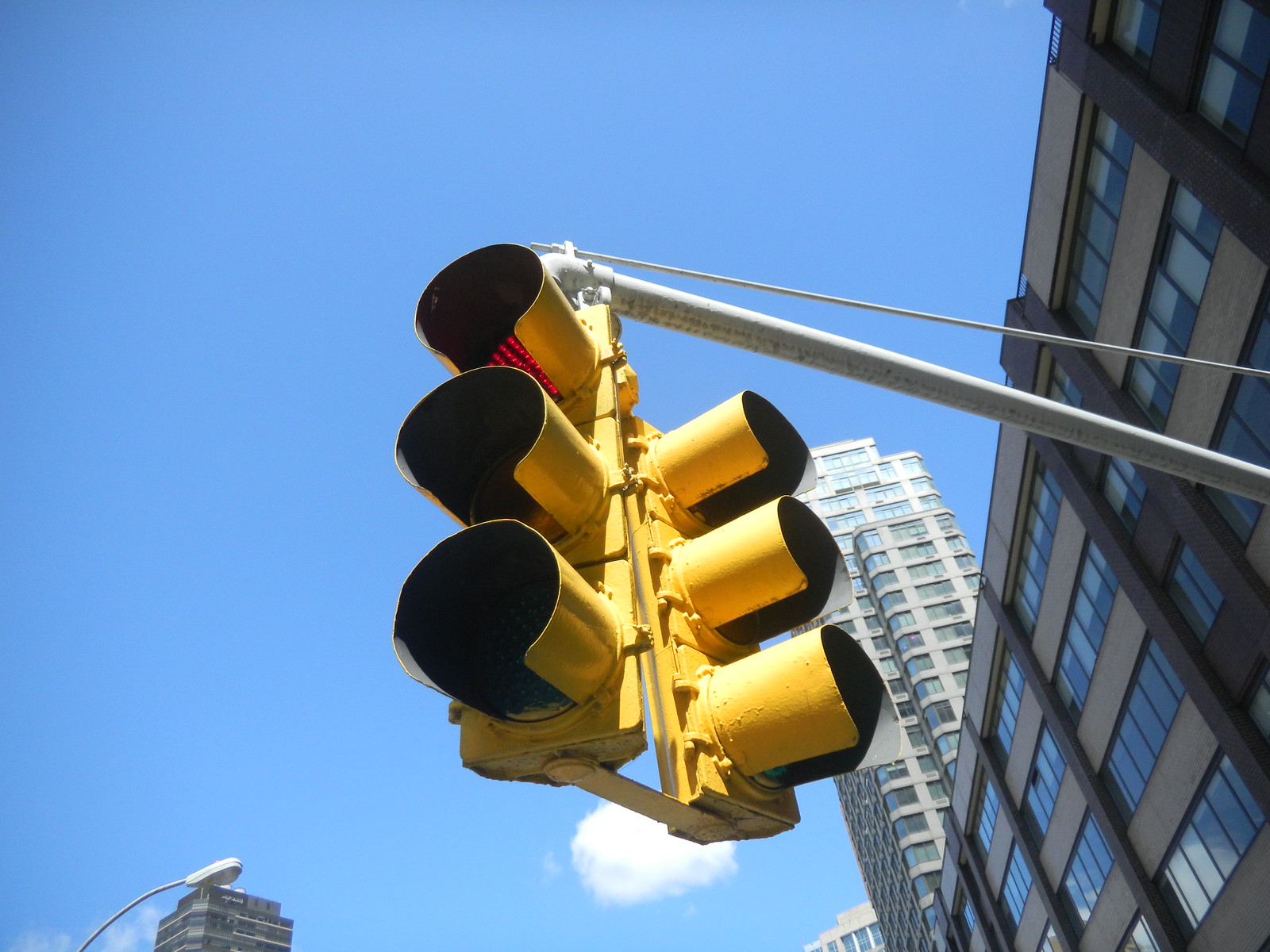In a bustling urban setting, two prominent yellow traffic lights are suspended from a metal pole, viewed from below at a close angle. The configuration shows one set of lights oriented directly towards the viewer, with its red light prominently lit, and the other set angled slightly to the right, showing a faintly visible green light. This distinctive viewpoint allows us to peer into the interior holes of each traffic light. The sky above is a vivid blue with a singular small cloud positioned under the intersection of the traffic lights. Surrounding this scene are a mix of towering skyscrapers and medium-sized buildings. To the right, a notable shorter building with at least four or five floors features a façade of brown sides with contrasting dark brown vertical and light brown horizontal trims, punctuated by numerous windows. Behind it stands a taller structure with light gray walls and several windows. On the left side, a small part of another tall building is visible along with a single unlit streetlight. The overall clarity of the sky and the lighting suggests that the image was captured on a sunny day at midday.